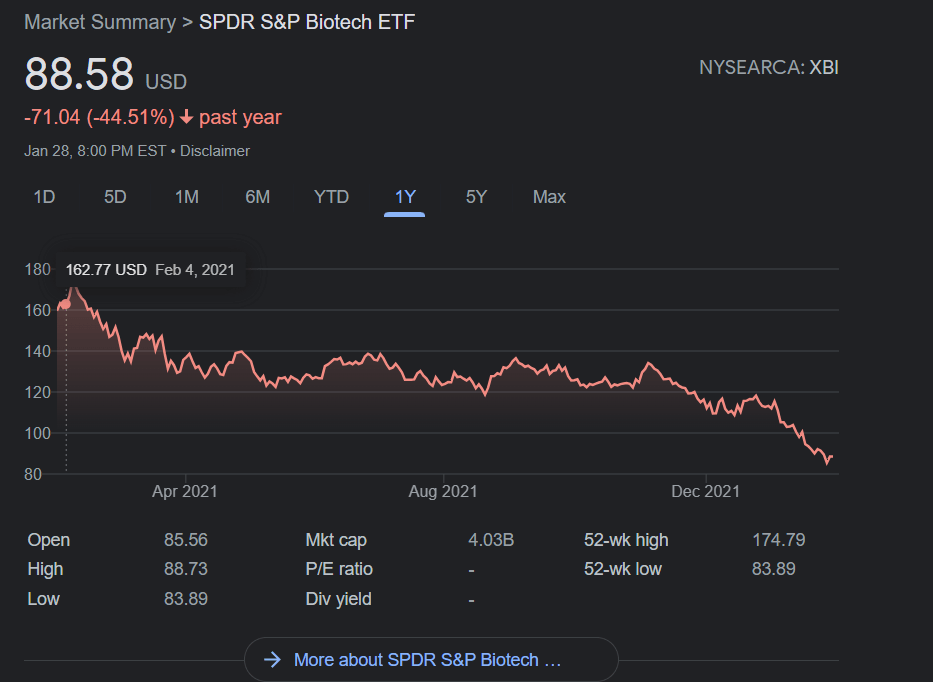Screenshot of a financial summary for the SPDR S&P Biotech ETF (XBI). The background is a combination of black and light gray tones. In the top left corner, the title "Market Summary" is displayed. Below it, there is a forward arrow followed by "SPDR S&P Biotech ETF". A label shows the current price as "88.58 USD".

On the right-hand side, the label "NYSERCA: XBI" is prominently featured. Beneath the price, in red, it indicates a significant decrease of "−71.04 (−44.51%)", accompanied by a red arrow pointing downwards indicating the past year's performance. The date and time "January 28th, 8 p.m. EST" along with a disclaimer in light gray are placed below this information.

A series of time frame options are listed: "1D, 5D, 1M, 6M, YTD, 1Y, 5Y, MAX". A graph below these options depicts a downward trend for the stock over approximately six months.

Further details are provided below the graph:
- Open: "85.56"
- High: "88.73"
- Low: "83.89"
- Market Cap: "4.03B"
- PE Ratio: "N/A"
- Div Yield: "N/A"
- 52 Week High: "174.79"
- 52 Week Low: "83.89"

At the very bottom, there is a blue arrow pointing to the right, labeled "More about SPDR S&P Biotech," which appears to be a clickable button for additional information.